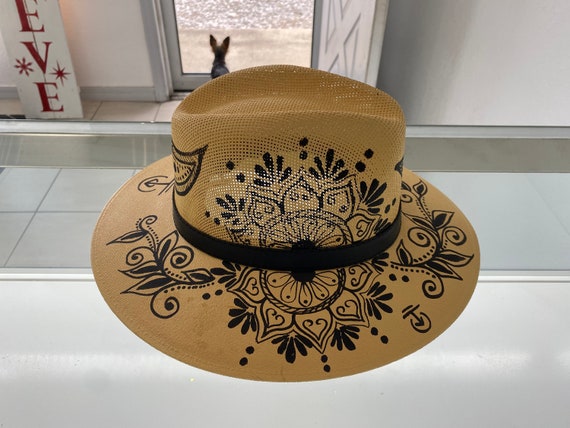In the photograph, a tan brim-style hat, reminiscent of a cowboy hat but with a distinctive flair, is prominently displayed. The hat features intricate black floral patterns, adding an elegant touch to its classic design. Encircling the base of the hat is a sleek black leather band, which complements the overall aesthetic. The hat is placed atop a white tiled countertop, which stands out against the neutral tones of the hat. In the background, the white wall portion merges seamlessly with the countertop. Further back, the scene reveals a tiled floor and a silhouette of a dog gazing out through a glass door. To the right of the dog, a white door stands ajar, while a small sign to the left reads "Eve" in red letters against a white backdrop.